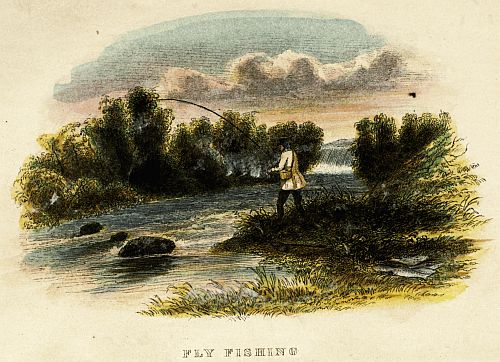This image resembles a vintage postcard or a drawing that could have appeared in a 1920s fly-fishing magazine, characterized by its age-related yellowing and fragile-looking paper stock. The picture is centralized within a circular frame, with the surrounding corners left bare. Rendered in a somewhat boxy font at the bottom, the words "fly fishing" are prominently displayed.

The scenery depicts a tranquil, yet dynamic setting with a blue sky painted with slightly darkened clouds, which might suggest the approach of evening. The picture features a rushing river, not too deep, with visible rocks and a cascade that appears to be a waterfall in the background. The riverbank where the fisherman stands is encircled by lush greenery, including tall trees, shrubs, and perhaps cattails in yellow-green hues behind him.

The central figure is a British-looking fly fisherman, donning a white jacket and armed with a large, bent fishing pole. He has a basket strapped around his body for holding his catch, with a few fish already laid out on the grassy riverbank beside him. The meticulous illustration also includes small birds adding to the serene and picturesque ambiance.